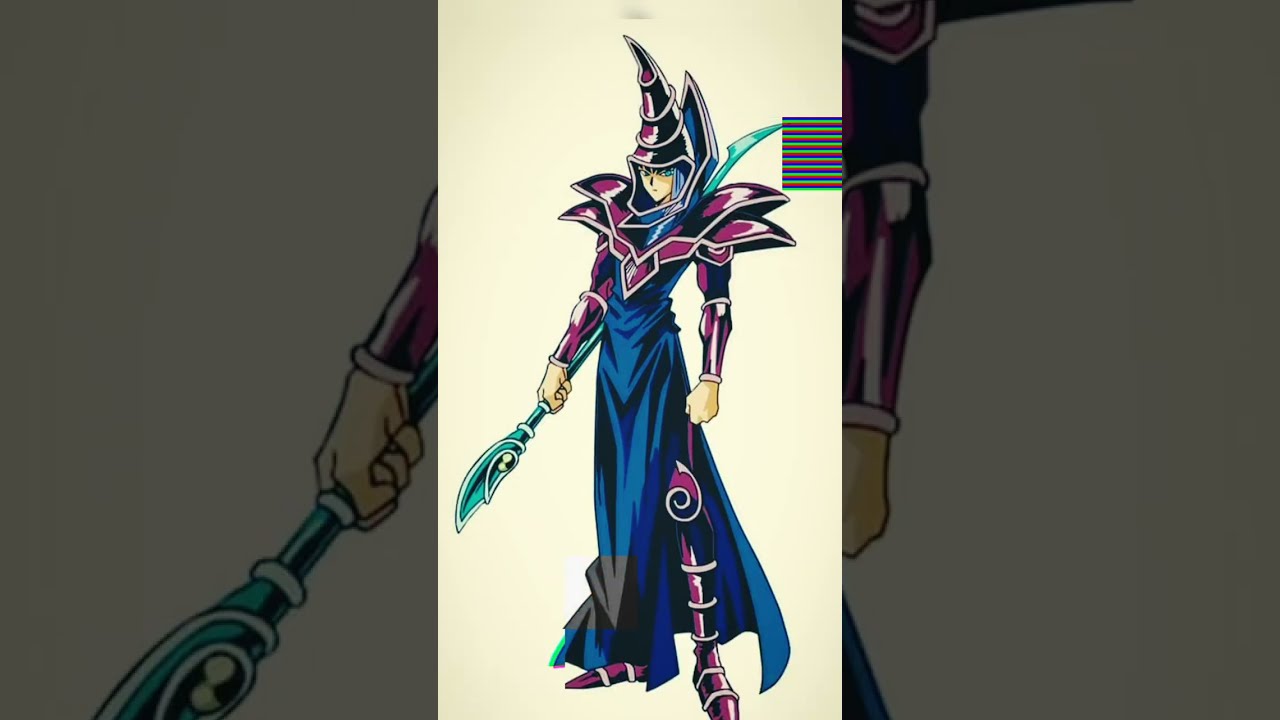The image showcases a detailed graphic design resembling a character from Yu-Gi-Oh in a manga or anime style. The central figure, prominently displayed in a vertical banner, is a wizard-like character with blue hair, partially concealed by a pointed helmet that is purplish-black in color. He wears a flowing blue robe paired with intricate metallic armor, including shoulder pads, armguards, and boots all matching the purplish hue of his helmet. In one hand, he holds a light blue or teal staff. The background features a light yellow, almost paper-like texture, with a shadowy close-up of the central figure creating a striking overlay effect. There are also faint stripes visible at the top right, adding to the intricate fantasy aesthetic of the design.